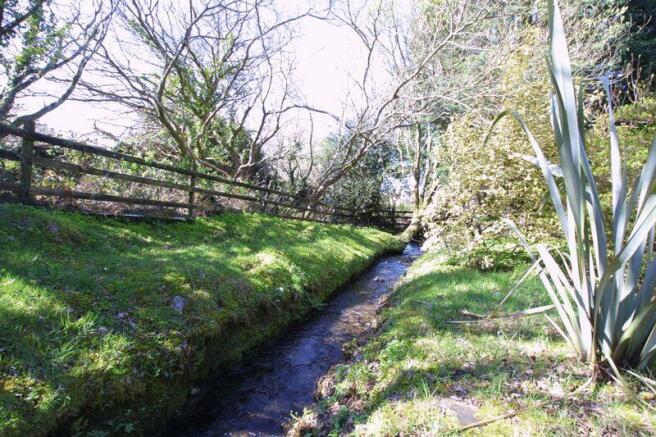In this outdoor nature setting, a small, narrow stream flows from the bottom to the middle right of the image, meandering through patches of grass-covered banks. On the left bank, a gentle hill slopes upward to a wooden rail fence with three widely spaced rails. Behind the fence, there are several dry, deciduous trees with bare branches. In contrast, the right bank features a prominent plant with long, lanceate leaves resembling ornamental flax, standing tall near the front of the image. Behind this plant, a mix of other green-leaved trees are visible. The serene scene is capped by a partly cloudy, whitish-blue sky, casting a gentle light over the tranquil landscape.